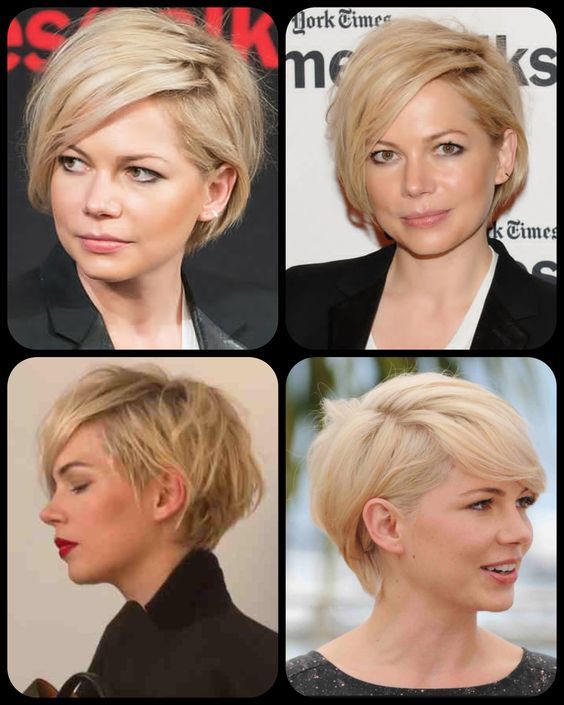The image features a collection of four distinct photographs of Michelle Williams, each positioned in the corners of the frame and showcasing her signature pixie cut hairstyle. The background prominently displays text that includes the words "New York Times," though some of the details are indistinguishable.

In the top left corner, Michelle Williams is seen with her pixie cut combed to one side, looking off to the right. The top right image captures her at an event, standing against a backdrop featuring "New York Times." In this photo, she gazes directly at the camera, her expression softened by a slight smile. 

The bottom left corner portrays her with eyes closed, head turned to the left, and her pixie cut slightly tousled for a stylish effect. Finally, in the bottom right corner, she smiles gently while looking to the left, her hair combed smoother than in the other images.

The collection’s colors include various shades of blonde, light blonde, red, pink, gray, green, white, and black, providing a diverse and vibrant visual palette that accentuates Michelle Williams in each distinct pose and setting.